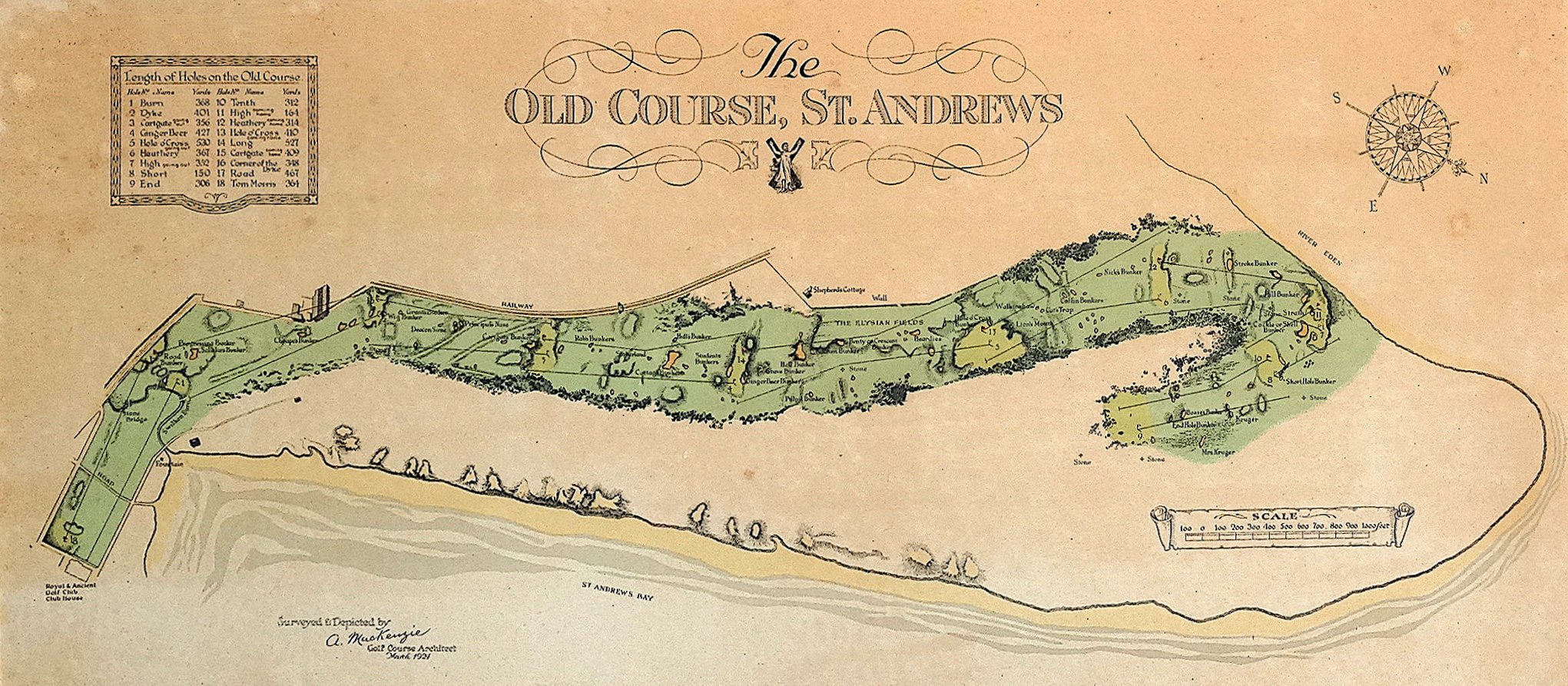This image is an old, detailed map of the St. Andrews Golf Course, depicted on aged parchment paper. At the top, the title "The Old Course St. Andrews" is prominently displayed in a combination of ornate cursive and old-world serif fonts, surrounded by decorative, swirly ornamentation in each corner. The map features a horizontal layout of the golf course, illustrated with black lines and lettering. The fairways and putting greens are painted in various shades of green, with lighter greens indicating the putting areas. Yellow shades accentuate particular regions, and tree lines, pathways, and the coastline are clearly marked. A compass in the upper right corner indicates directions, with north pointing down-right. In the top left corner, a legend titled "Length of Holes on the Old Course," details the course layout from hole 1 to 18. The map's scale is located in the bottom right corner. The course's description reflects a Lynx style, with the St. Andrews Bay depicted along the bottom edge, emphasizing its coastal setting.